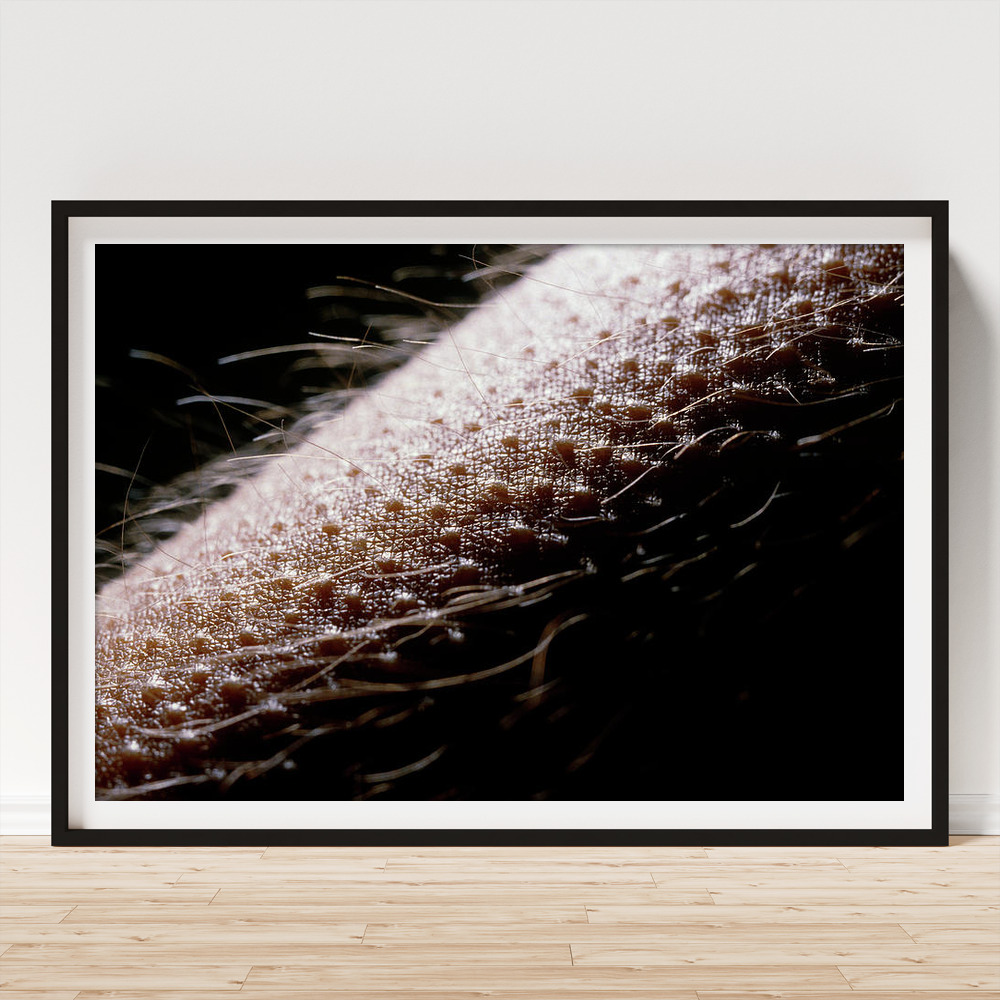The image depicts a digitally altered stock photo of a framed art print, set against a minimalist backdrop. The black-framed and white-matted picture rests on a light brown wooden floor, leaning against a white wall with a white baseboard. The framed photo is an extreme close-up of skin, showcasing detailed textures, pores, and goosebumps, with fine hairs standing on end from each raised bump. The high-contrast image, predominantly in shades of black and nearly white, is illuminated by light coming from the top-left corner, highlighting the intricate patterns and giving it a dramatic, almost monochromatic appearance.